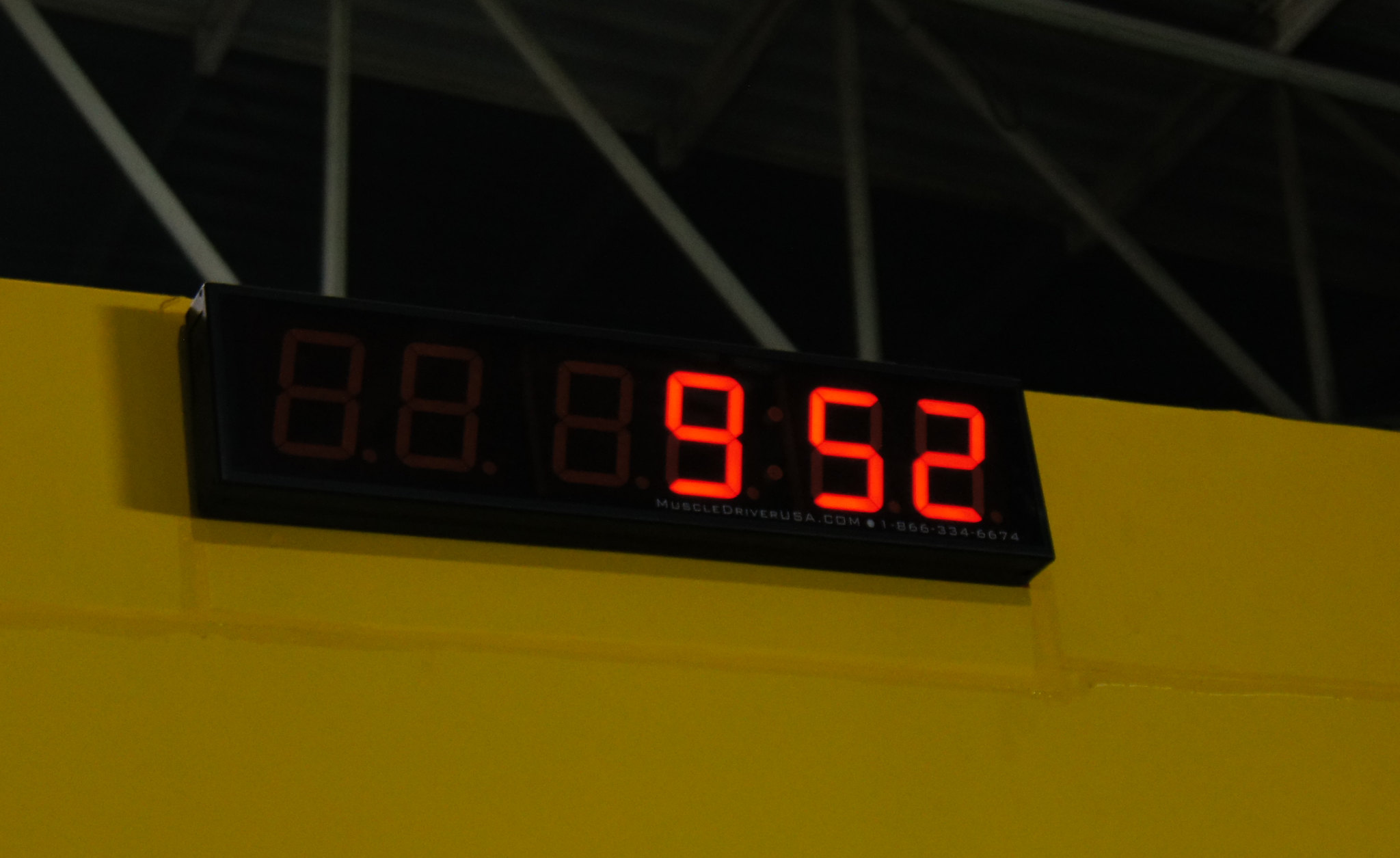The image depicts a large black LED clock displaying the numbers "952" in bright red. It is mounted on a vibrant yellow wall, giving a stark contrast to the clock's black casing. The setting appears to be a gymnasium or train station, suggested by the presence of silver steel girders visible above the clock. The red LED numbers are clearly illuminated, and beneath the clock, the text "MuscleDriverUSA.com" is visible, along with the phone number "1-866-334-6674." The overall scene is striking with its vivid color contrasts and structural elements, emphasizing the gym-like atmosphere.